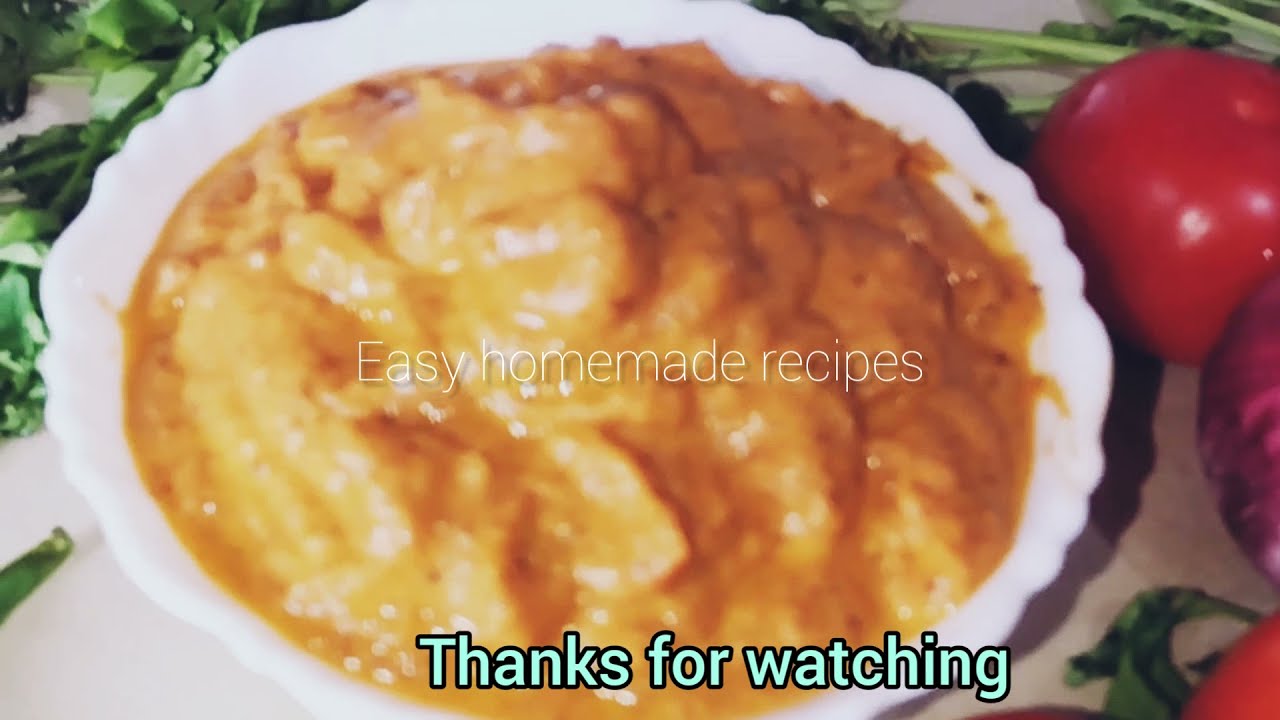This image highlights a white scalloped bowl filled nearly to the brim with a thick, yellowish liquid paste, possibly porridge or mashed potatoes, topped with a shiny brown gravy. Positioned on a white table, the bowl is surrounded by various scattered vegetables: leafy greens in the upper left corner, a whole tomato, and a partially visible purple onion. The photo features superimposed white text across the middle of the bowl, reading "Easy Homemade Recipes," while the bottom edge displays bolder text that says "Thanks for Watching," suggesting the image might be associated with a food vlog, TV show, or live stream about cooking.